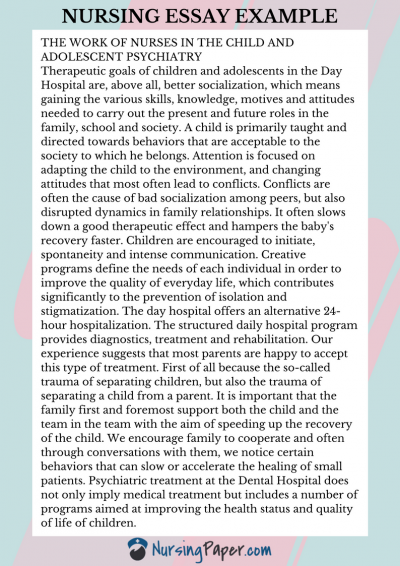**Nursing Essay Example**

The backdrop of this digital image features a serene, pastel color scheme with a primarily light greenish-blue hue, interspersed with delicate pink and lavender splotches. The top of the image prominently displays the title, "NURSING ESSAY EXAMPLE," in bold, all-caps serif font. 

At the bottom, "Nursing Paper dot com" is written in a handwritten style font, where "Nursing" and "dot com" appear in blue, while "Paper" is in black. To the left of this text is a logo depicting a dark gray silhouette of a mountain crowned with a blue nurse's hat.

Spanning the vertical space between the title and the logo, a white rectangle with a light gray background contains the essay's opening segment. It begins with an all-caps black header that states, "THE WORK OF NURSES IN CHILD AND ADOLESCENT PSYCHIATRY."

Beneath the header lies the introductory paragraph, detailing the therapeutic goals in a day hospital setting for children and adolescents. It describes the overarching aim of better socialization, encompassing the acquisition of skills, knowledge, motives, and attitudes essential for familial, educational, and societal roles. Emphasis is placed on behavioral modification to align with societal expectations, environmental adaptation, and attitude adjustments to mitigate conflicts—often the root of poor peer socialization and disruptive family dynamics. These factors can decelerate therapeutic progress and recovery. Children are encouraged towards spontaneity and robust communication, with creative programs tailored to meet individual needs, enhancing the quality of daily life.

The paragraph continues in a similar explanatory tone, elaborating on these themes.